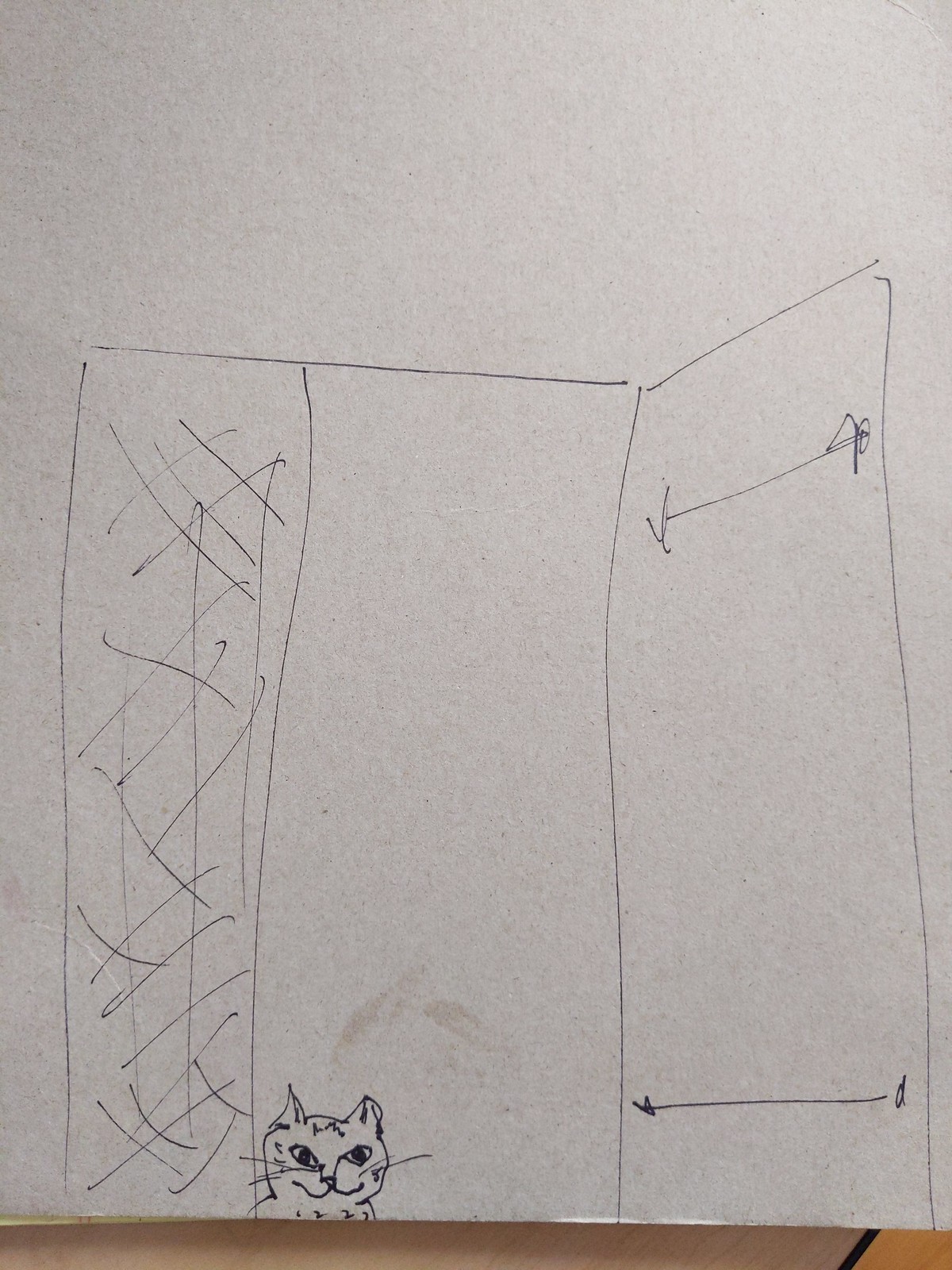A finely detailed black fineliner drawing is presented on a piece of white paper, which seems to have a textured surface akin to that of sketchbook paper under the influence of lighting. At the bottom of the photograph, the edge of the paper reveals a beige surface beneath, with a part in the bottom right corner showing a more orangish tint, reminiscent of a pine floor. The centerpiece of the drawing features an open window, framed on the left by sketched curtains. The nature of the window itself remains ambiguous; it could be either the windowpane or a shutter, identifiable only as a rectangle with two horizontal lines bisecting it. At the bottom of the window, intricately drawn in contrast with the rest of the sketch, is the head of a grinning cat, complete with detailed eyes, whiskers, and fur markings, suggesting the artist invested significantly more effort in rendering the feline culprit.